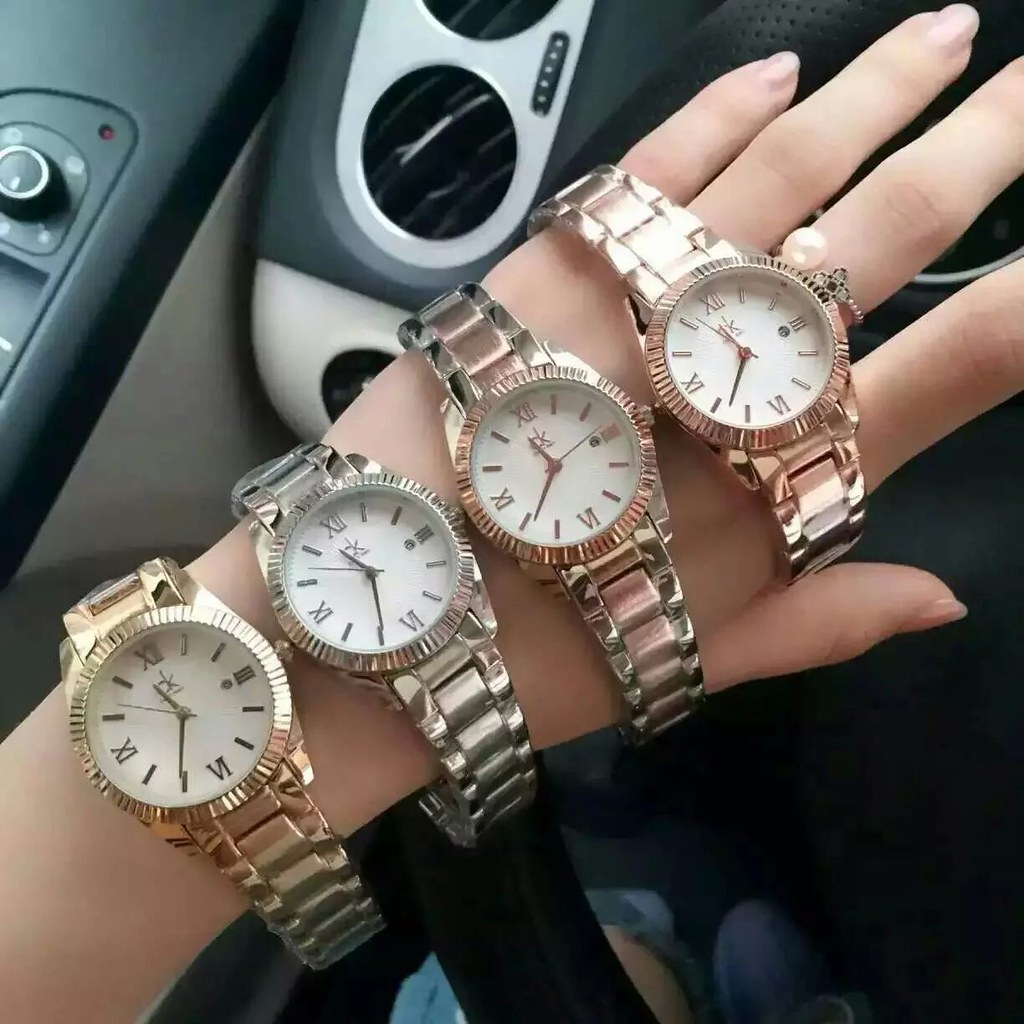The photograph, in a square orientation, captures the top view of a left hand extending diagonally from the bottom left towards the top right. The hand, adorned with light pink nail polish, prominently displays four analogue wristwatches with off-white cream Roman numeral faces. Each watch features a metal strap; the two closest to the knuckles have a slightly worn, rose gold tint, suggesting wear over time. The other two feature golden and silver tones. The person appears to be seated inside a vehicle, as evidenced by the blurred background revealing elements of a car dashboard, including circular vents, a control knob, and possibly the person’s knee and blue trainer shoe. Additionally, a light ring is visible on the middle finger of the hand. The overall setting could either depict a real-life scenario or a staged product display for selling the wristwatches.